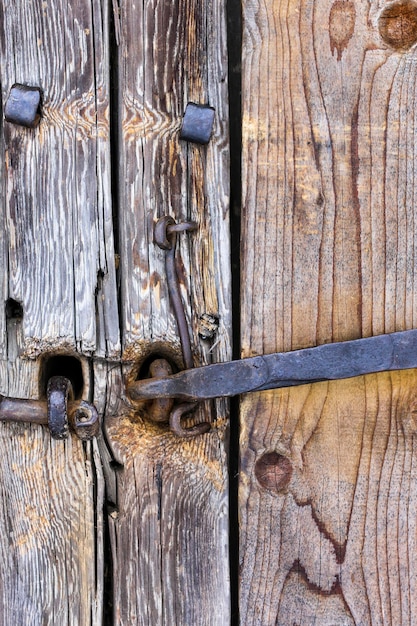This color photograph captures a close-up view of an old wooden gate, showcasing three vertical wooden posts with varying thicknesses. The post on the left extends beyond the frame, while the middle post is thinner, and the right post is thicker, also extending beyond the frame. The weathered wood, in shades of light and dark brown, appears slightly gray from age and exposure. 

At the top of the left and middle posts, small metal knobs are visible. Midway down the left post, there's a round metal piece with another cylindrical piece of metal extending horizontally and exiting the frame on the left. In the middle post, slightly above center, a small metal loop is present. A metal piece goes through this loop, extending downward and ending with a hook, suggesting a locking mechanism. Above this hook, another metal piece extends rightward and slightly upward, crossing over to the right post and out of the image.

The metal elements appear to be old wrought iron, possibly crafted by a blacksmith, evidenced by their oxidized black look but relatively rust-free appearance, indicating high-quality material. The configuration of metal loops, bars, and rivets implies a functional role in securing or binding the gate, blending rustic craftsmanship with utilitarian design.